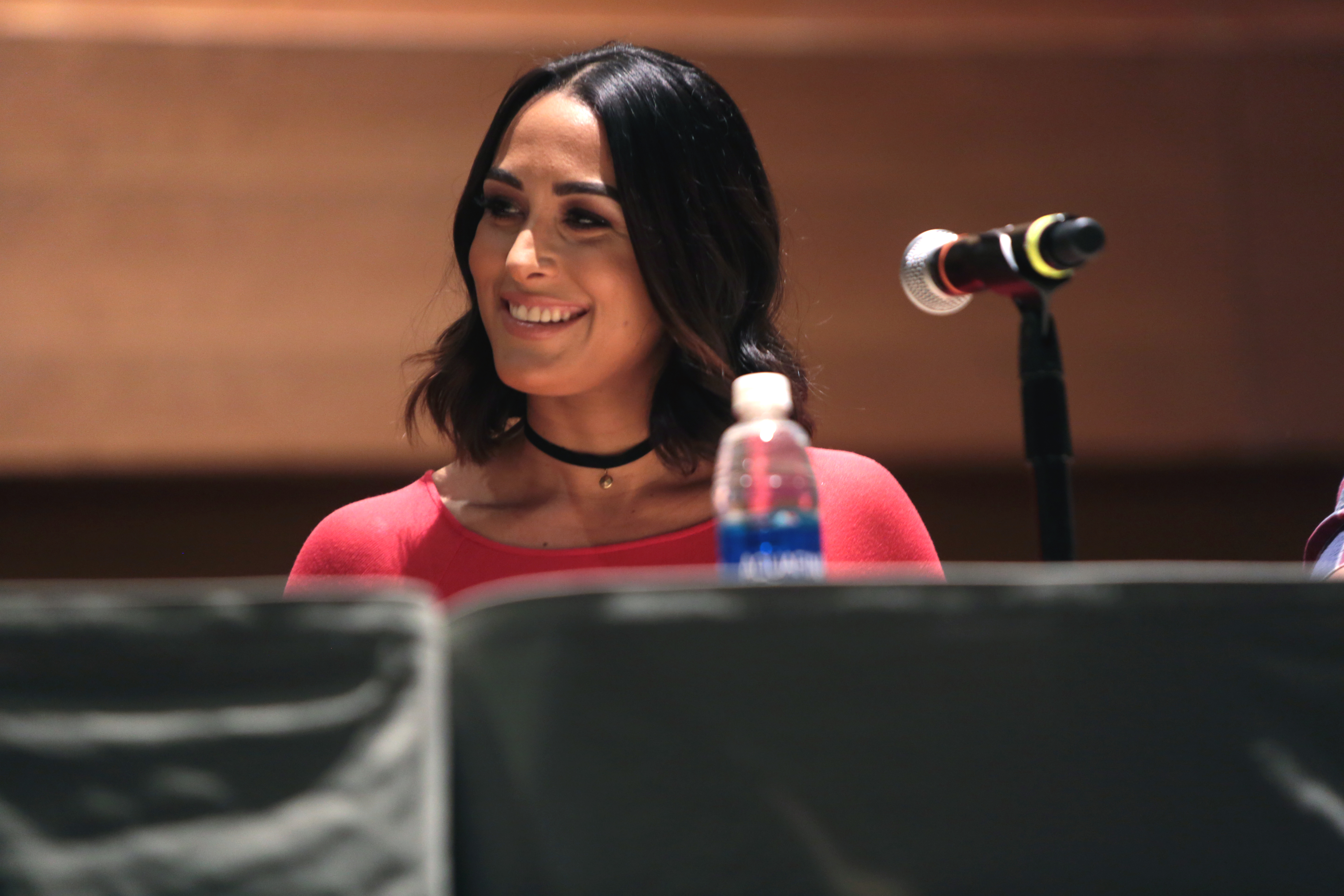The photograph depicts a young woman sitting behind a long table that spans the width of the image. The table has a gray covering which might be plastic or cloth. The woman, visible from the chest up, faces forward while her gaze is directed to the left, revealing her beautiful smile. She has shiny, shoulder-length, wavy dark hair, complemented by dark eyebrows and eyes. She is wearing a form-fitting, low-cut pink, possibly red, top. Around her neck is a black choker necklace with a gold pendant hanging from it. In front of her, on the table, there's a plastic water bottle slightly to her right. Further to the right, there's a microphone pointing towards her. The background is blurred, with a lighter top and a darker bottom, resembling a wall. The foreground also features two out-of-focus gray rectangular shapes, possibly the backs of chairs.